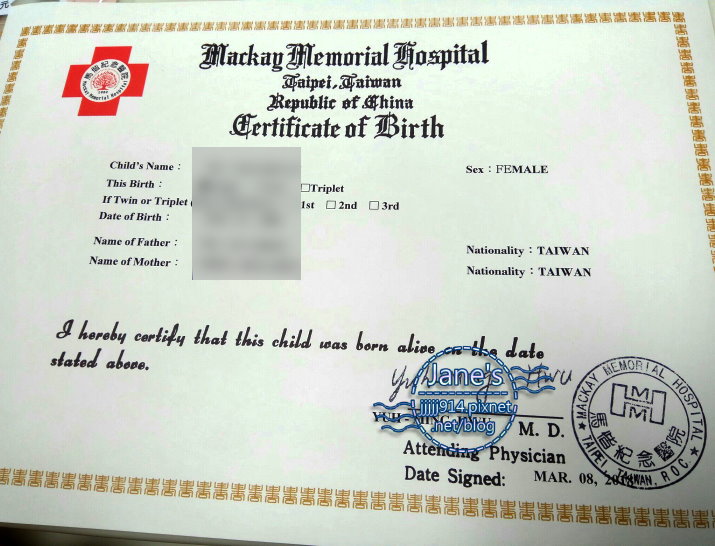The image displays a rectangular birth certificate with a gold border, issued by MacKay Memorial Hospital in Taipei, Taiwan, Republic of China. The certificate features black text on a white background with the title "Certificate of Birth" prominently centered at the top. In the upper left corner, there is a red cross with a red tree symbol inside a circle, accompanied by the hospital's name. The document includes fields for the child's name, sex, date of birth, whether the child is a twin or triplet, and the names and nationalities of the mother and father, all of which are blurred to protect privacy. It also includes a statement certifying that the child was born alive on the specified date, alongside the physician's stamp, signature, and date signed. Red seals or stamps are present, adding to the document's authenticity. Additionally, an overlay in blue text with a circular border advertises "Jane's JJJ914PixNet.net/blog."